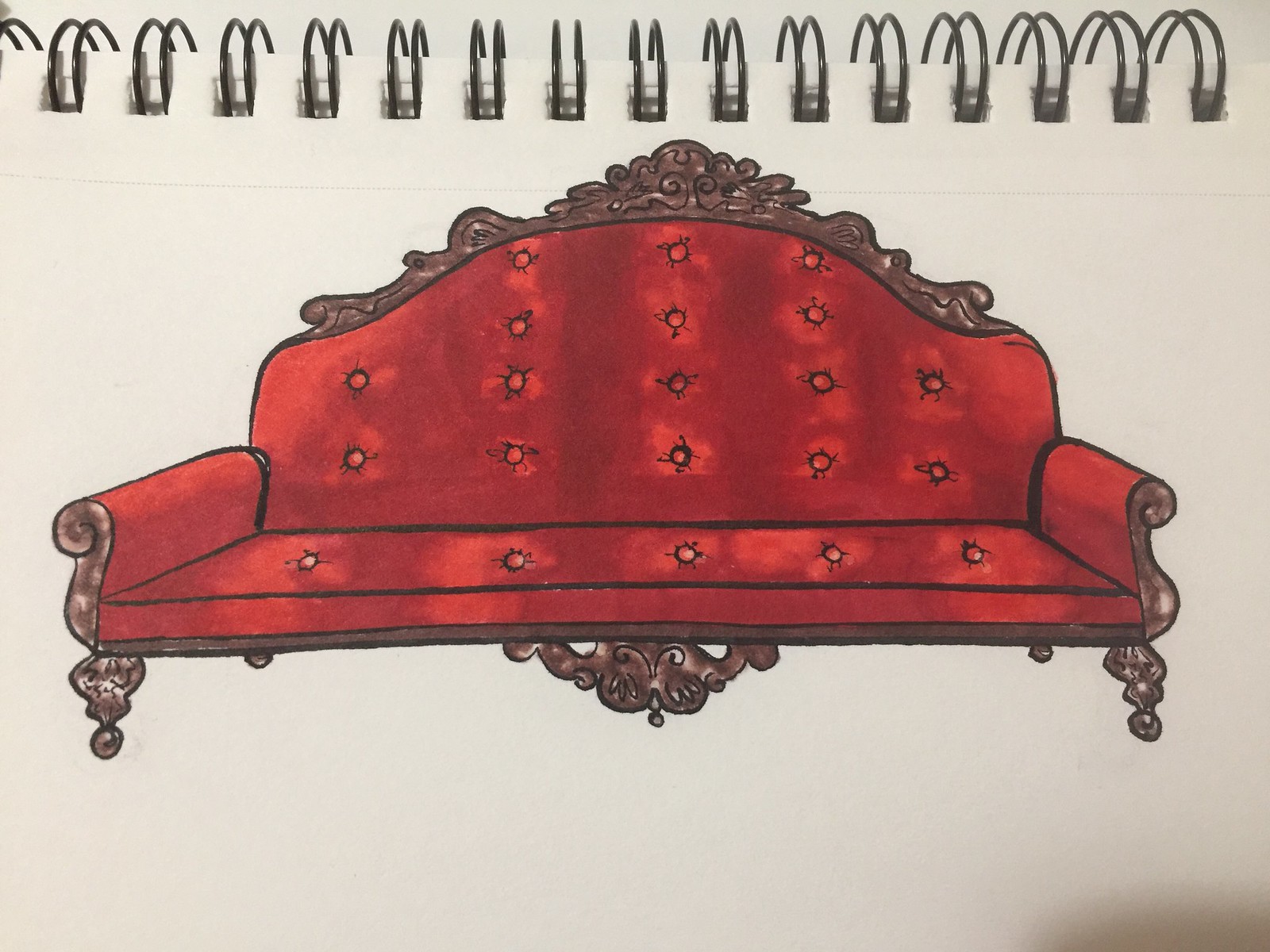The image depicts a luxurious dark red velvet settee positioned on a blank piece of white paper, which appears to be taken from a spiral notebook, evident by the visible spirals at the top of the page. The settee is adorned with intricate tufting, featuring button detailing—three buttons on each side and a central column of five, with four on the backrest and one on the single seat cushion. The side armrests are also covered in the same deep red velvet fabric. Adding to its elegance are ornate metal filigree decorations that curve gracefully at the top of the settee and are also evident in the middle of the bottom section. The settee is supported by four exquisitely detailed legs, completing its sophisticated appearance.